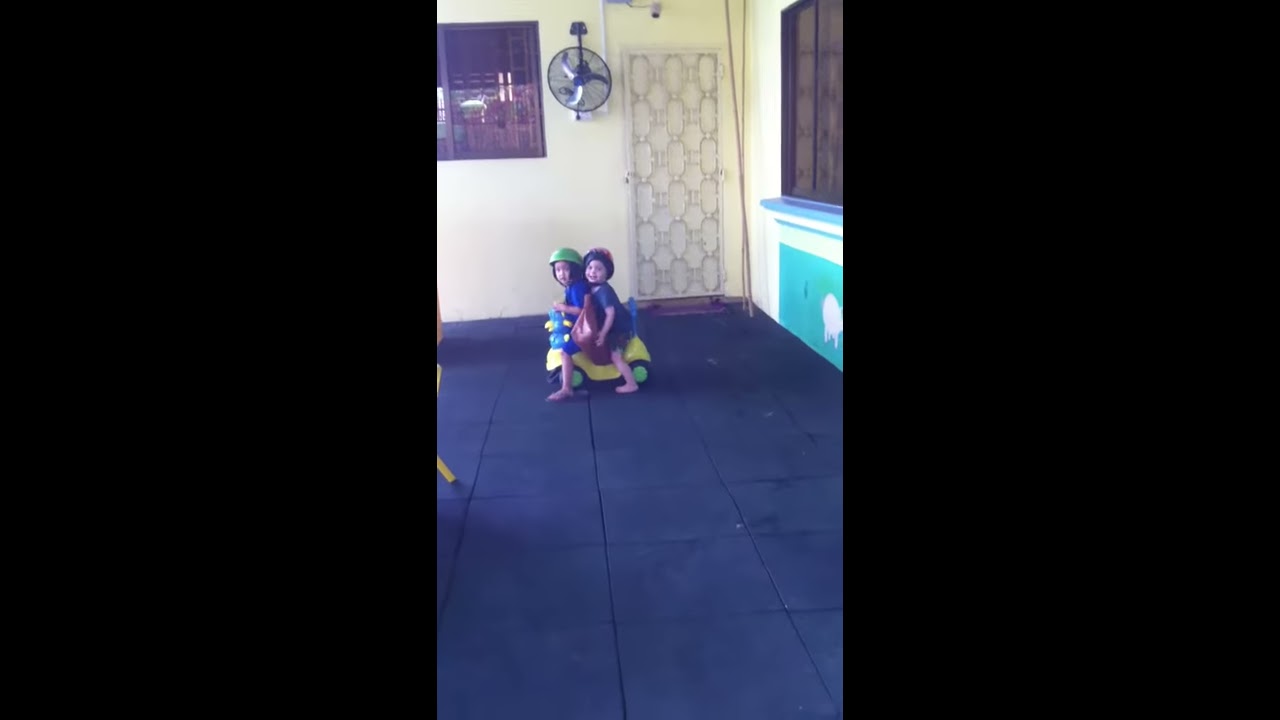This is a casual photographic image capturing a pair of toddlers, presumably Asian, indoors in a room with vibrant yellow walls and soft black square tiles on the floor, ideal for children's play. They are seated on a small yellow plastic vehicle with green wheels, which seems designed for one but accommodates both children. The child in front wears a green helmet, and both children are dressed in blue shirts. One child, potentially wearing sandals or barefoot, has an item reminiscent of a hairband. 

In the background, a wall-mounted fan is visible above the children, hinting at a playroom or a home environment. To the right, there are a couple of windows indicated in the scene, and at least one of them shows it's night outside. There's some brown paneling and possibly a door or additional wall features. Notably, a bag is situated between the children on the toy. The amalgamation of these elements paints an intricate depiction of their playful indoor setting.